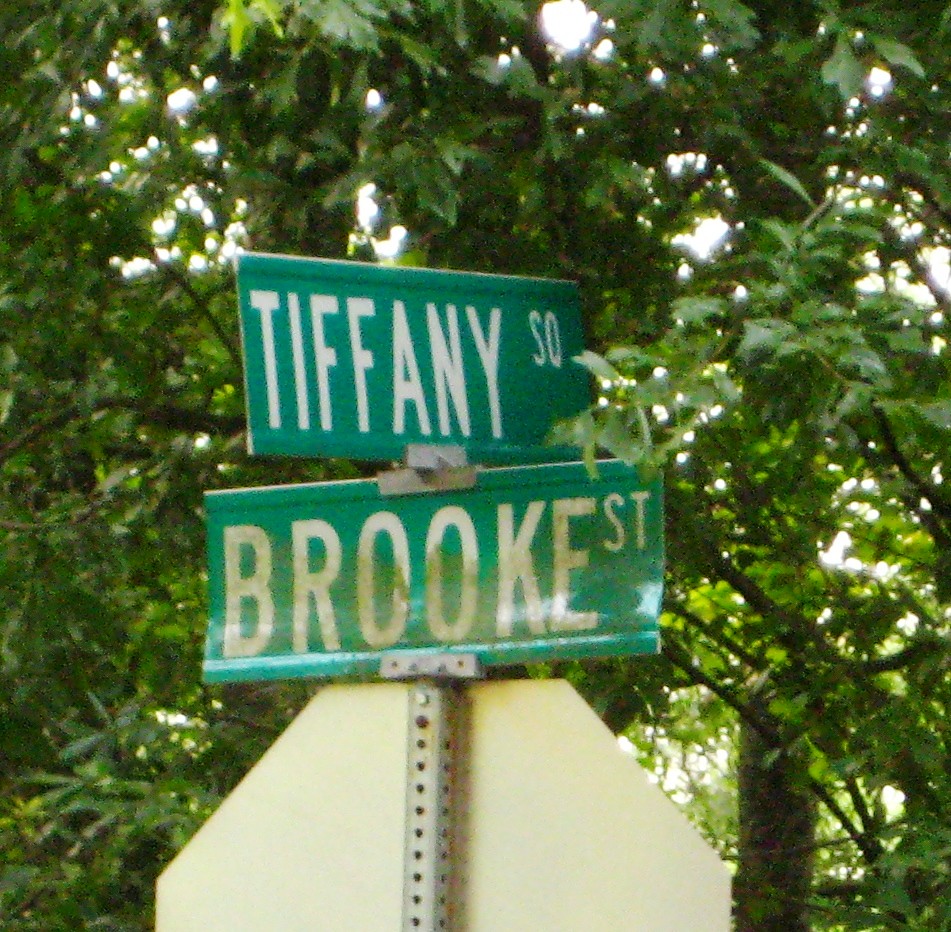The image captures a lush backdrop of vibrant green foliage with glimpses of sunlight filtering through, creating pockets of bright white light amidst the leaves. The dense greenery is interspersed with tree trunks rising through the foliage. Prominently featured in the foreground are two green street signs mounted on a silver post with multiple black holes. The top sign reads "Tiffany S.O." in bold white text, pointing to the right. Below it, a dirt-smudged sign reading "Brooke Street" in white text points to the left. Both signs are arranged perpendicularly. Just below them, the back of a stop sign is visible, delineated by its characteristic white half-octagon shape.